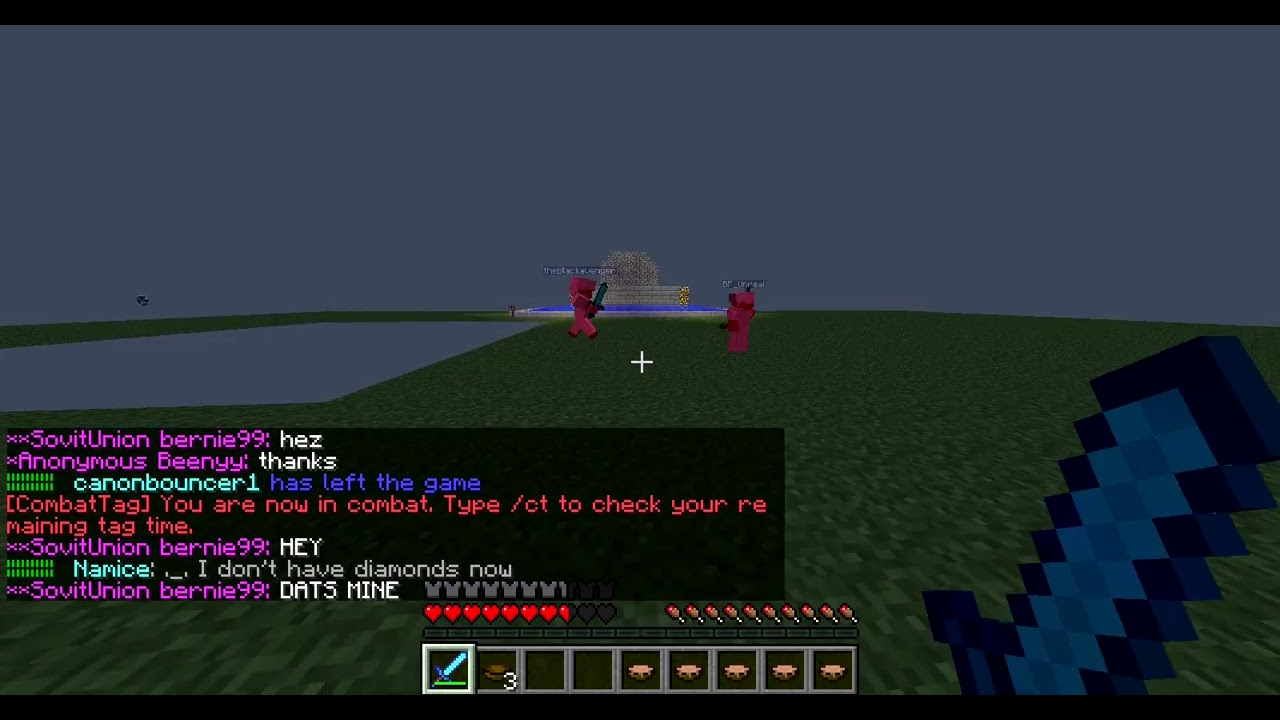The screenshot captures a pixelated scene from the PC game Minecraft. The backdrop features a grayish dark background with a grassy green foreground, illustrating the game's characteristic blocky style. Centrally, two diminutive, pink-clad characters are depicted from a top-down perspective. The character on the left grips a green sword, seemingly engaging with the other, who stands passively. Behind the sword-wielding character, there's a gray, blank patch. On the lower right corner, parts of a dark blue and light blue two-dimensional tower are faintly visible.

Towards the bottom left, a plethora of text occupies a grayed-out bar, displaying colorful dialogue: "Soviet Union, Bernie 99: HEZ," followed by "anonymous beanie, thanks," and "cannon bouncer one has left the game (Combat Tag) You are now in combat type /CT to check your main tag time." The chat continues with "Soviet Union, Bernie 99: hey name is... I don’t have diamonds now," and "Soviet Union, Bernie 99: that's mine." Heart emojis and various other small icons pepper the lower section of the screen. Thin black bars frame the top and bottom edges of the image, confirming its status as a digital screenshot of an in-game moment.